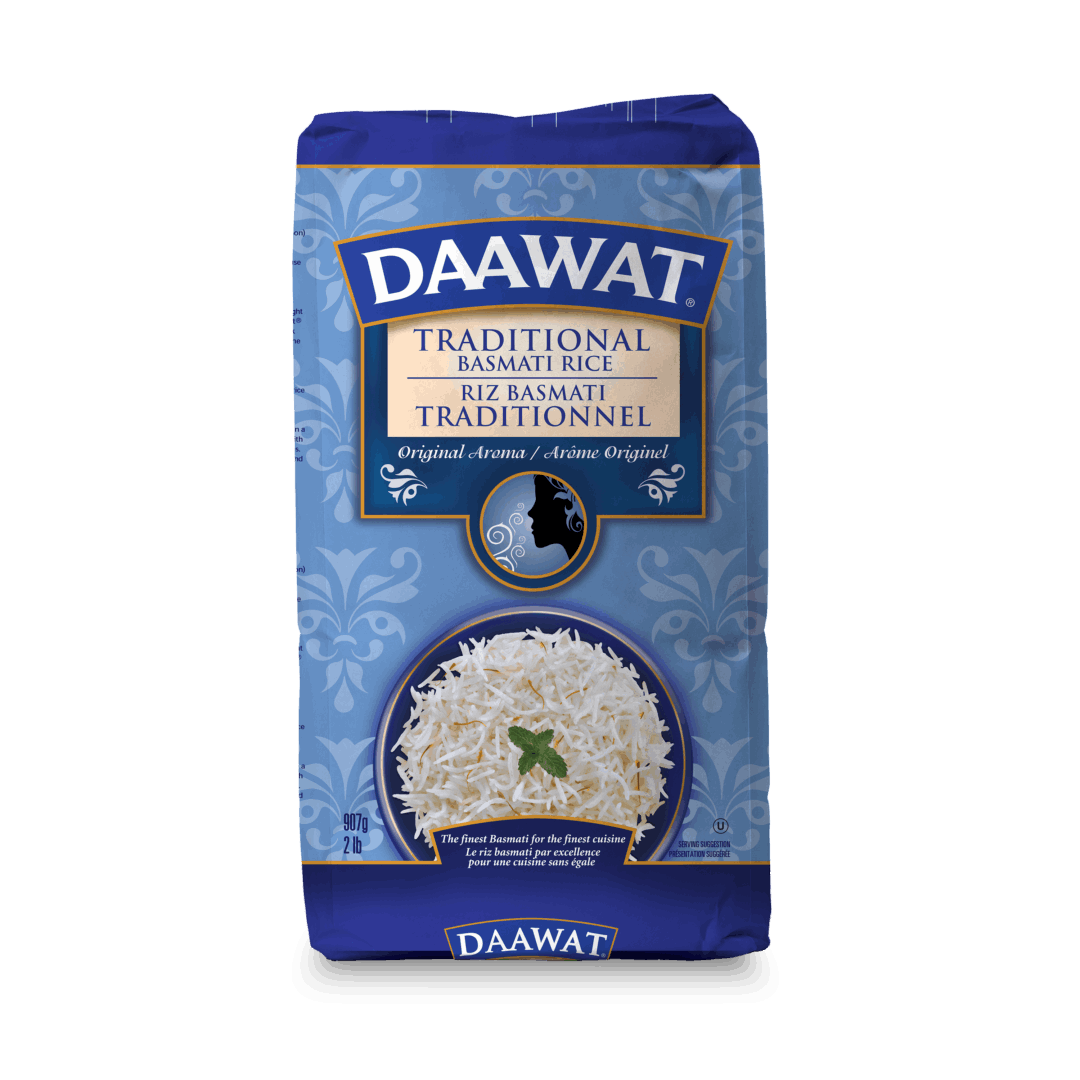The image showcases a close-up view of a rectangular bag of Dawat Traditional Basmati Rice, set against a solid white background. The visually striking bag features a two-tone blue color scheme: a dark rich blue at the top and bottom, and a lighter grayish-blue center adorned with white ornate floral decorations. Prominently displayed in white text is "Dawat Traditional Basmati Rice, Riz Basmati Traditionnel, Original, Aroma, Arome," underscoring its authentic flavor. Central to the design is an evocative graphic— a silhouette of a person experiencing the aroma of the rice, illustrated with gentle fumes rising towards their face. Below this graphic sits an inviting image of a bowl filled with Basmati rice, garnished with what appears to be a mint leaf, presented on a blue plate. Once again, at the bottom of the bag, the name "Dawat" is reiterated in bold white text.